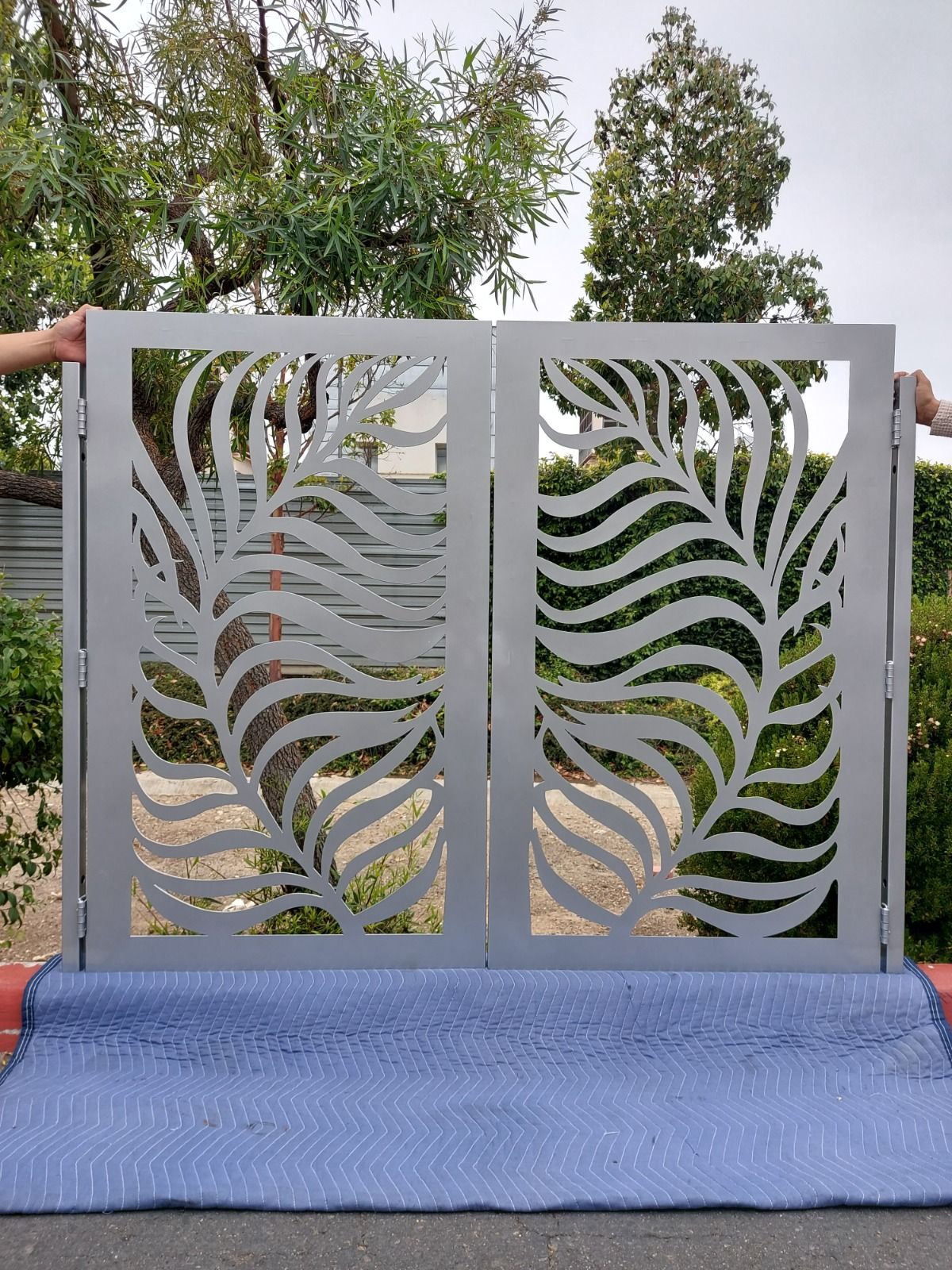This color photograph captures a detailed scene of a white metal gate placed on a light blue padded moving blanket with darker blue edges, commonly used with U-Haul trucks. The gate, appearing temporarily positioned and held upright by human hands on either side, features an intricate design with cutouts shaped like broad leaves, where the veins and curves of the leaves create a visually arresting, lace-like pattern. In the background, an outdoor garden is visible, featuring small trees that resemble olive trees, several hedge bushes, some shrubbery, and a low brick wall. The scene is set under a blue sky, with a gray fence also present in the backdrop, adding to the picturesque and well-composed garden setting.